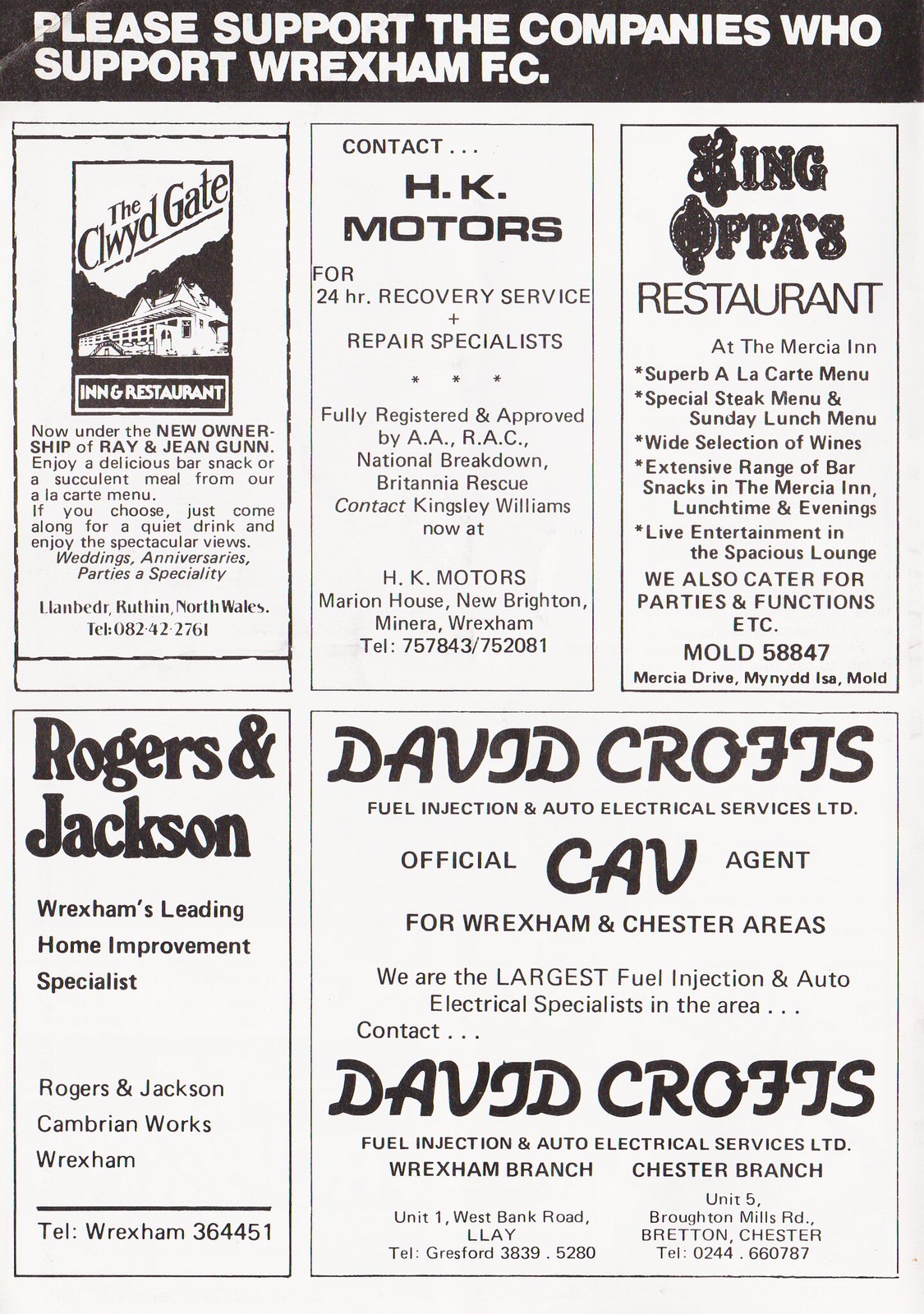The image depicts an aged, monochromatic poster or magazine page with a header that reads, "Please support the companies who support Rexham FC." The layout consists of five distinct rectangular ads. The first ad on the left is for the Clyde Gate Inn and Restaurant, which highlights services for weddings, anniversaries, and parties, mentioning their specialties in Lambert, Ruth, and Wales, along with their contact information. Adjacent to it is an ad for HK Motors, offering 24-hour recovery service and repair specialists, including their address and phone number. Next is an ad for King Offa's Restaurant with similar details, including contact information. Below is an ad for Rogers & Jackson, promoting them as Rexham’s leading home improvement specialists, with their phone number listed. Finally, the ad on the right is for David Croft's CAV Fuel Injection and Auto Electrical Services LTD, which provides their address, phone number, and specifies they are an official CAV agent. The poster's overall appearance suggests it dates back a few decades, with a clear, well-spaced design in shades of black, white, and gray.